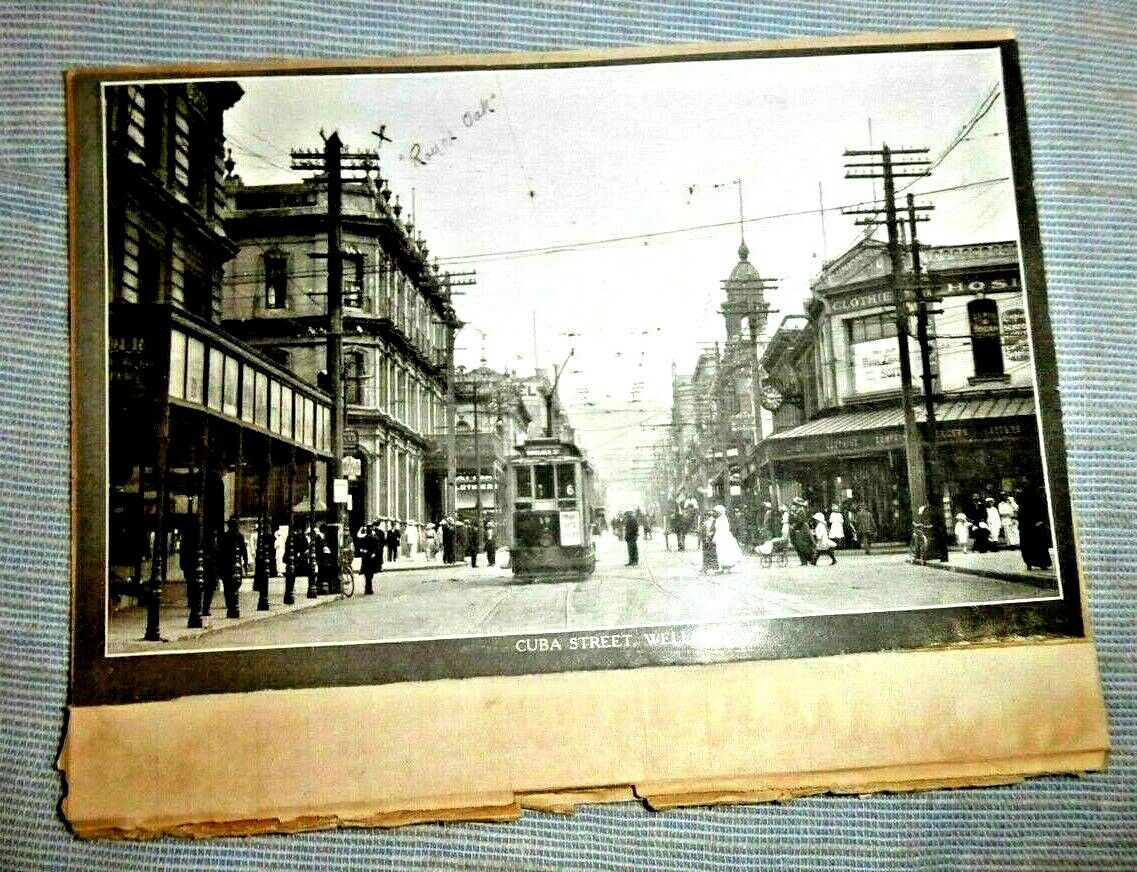This black-and-white photograph, bordered in black, appears to be an old image capturing a bustling downtown scene. At the bottom of the photograph, white writing clearly states "Cuba Street," followed by partially legible text, likely "Wellington." The center of the image features a prominent cable car marked with the number 6 on its front window, making its way down the street amidst a crowd of people walking about. Overhead, the sky is overcast, adding a cloudy ambiance to the daylight scene. Additional writing is visible on the upper left-hand side of the image, with the words "Royal Oak" discernible. The photograph, rich in historical essence, paints a vivid picture of a once thriving street filled with life and movement.